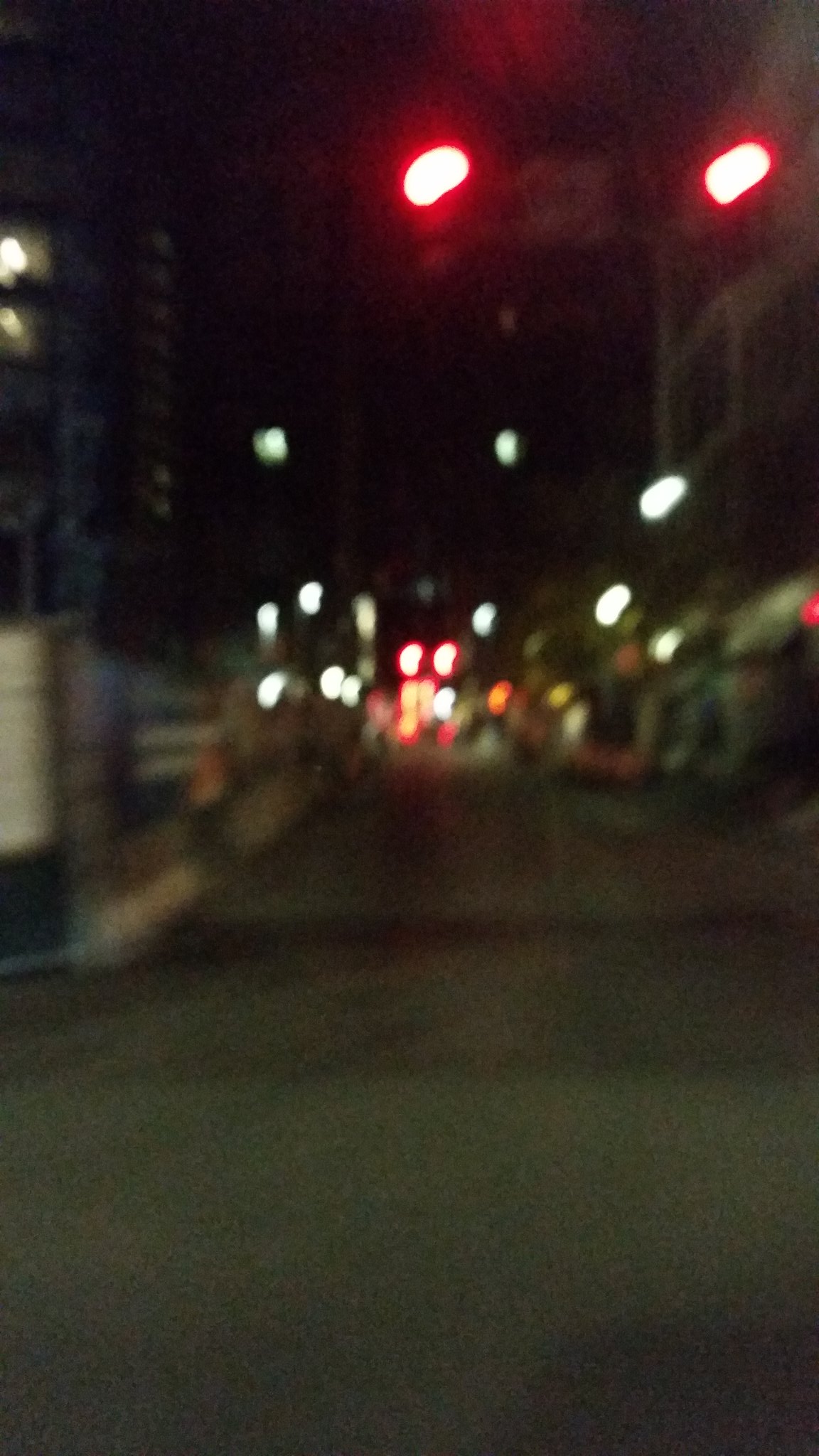The image portrays a dimly-lit, deserted street scene at night, shrouded in an intriguing blur. The view stretches down a seemingly long alley or suburban street, enveloped in shadows and mystery. Far in the distance, neon lights from shopfronts flicker, casting a faint glow that barely pierces the darkness. Overhead streetlights sporadically illuminate the path below, adding to the scene's eerie atmosphere. Dominating the top right corner are two prominent red lights, large and ambiguously close compared to the other lights in the image. Their purpose remains unclear, possibly belonging to a billboard or signpost, but the heavy blur renders them unreadable. The overall composition exudes an enigmatic quality, amplified by the absence of people and the indistinct details, evoking a sense of solitude and curiosity.